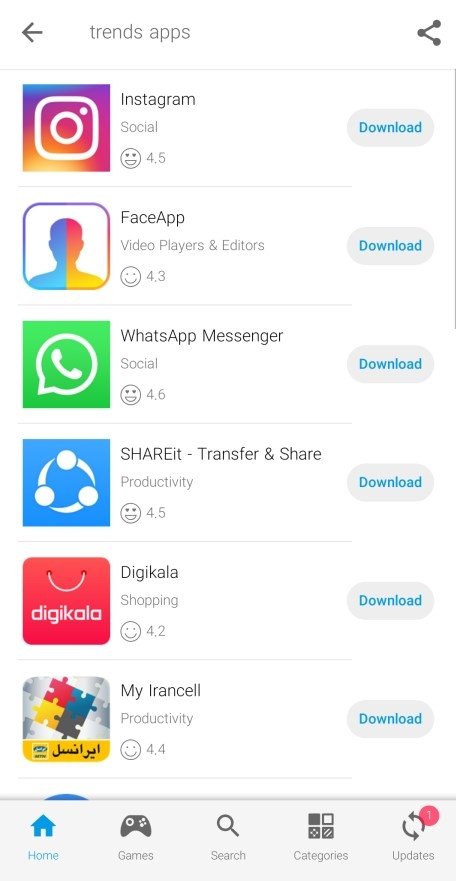The screenshot captures the interface of a mobile application trending and app listing page. The top of the screen includes a navigation option indicating the user is currently on the "Trends and Apps" section and has the ability to share the page. Below, a vertically scrollable list displays app logos, names, categories, ratings, and download buttons.

1. **Instagram**: Positioned under the header, this app is categorized under "Social" and features a happy face emoji. It boasts a solid 4 out of 5 stars rating.
2. **Face App**: Listed in the "Video Players and Editors" category with a 4.3-star rating and a smiley face emoji.
3. **WhatsApp Messenger**: This "Social" app is notably highly rated with a 4.6-star rating.
4. **Share It**: Falling under "Transfer and Share" for "Productivity", this app has an open-mouthed happy face and a 4.5-star rating.
5. **Digicayla**: A "Shopping" app, accompanied by a smiley face and a 4.2-star rating.
6. **My Arancel**: Featuring Arabic lettering, this "Productivity" app has a 4.4-star rating and a happy smiley face emoji.

Each app on the list has a download button to the right, providing users with easy access to the apps directly from this screen.